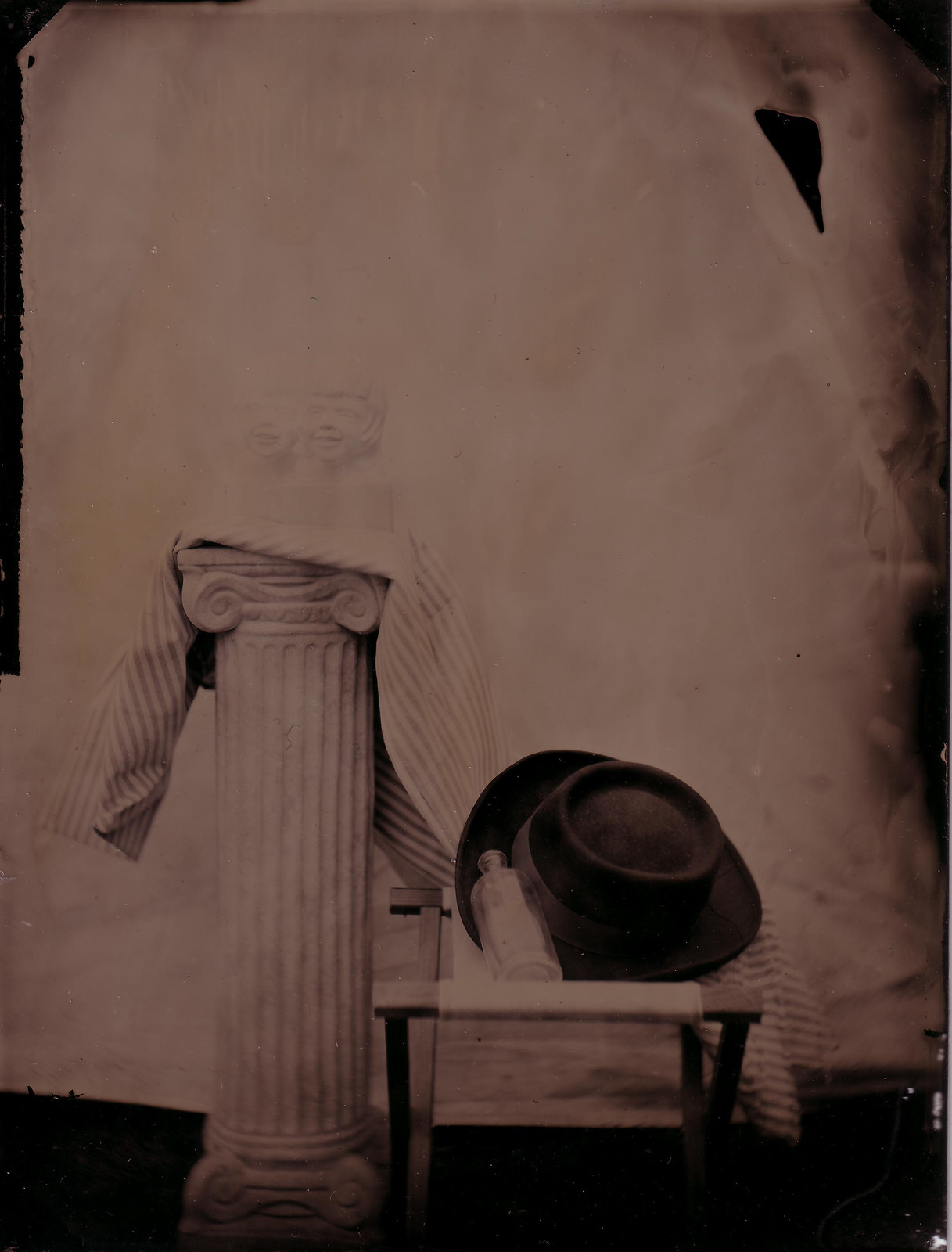The image appears to be an artistic black and white photograph evoking an older period, possibly the early to mid-20th century, given its vintage aesthetic. The composition features a prominent off-white Greek-style pedestal draped in a blanket or sheet, lending the scene a somewhat eerie, vintage atmosphere. Atop the pedestal and partially obscured by the drapery are two shadowy, statue-like faces of children, adding to the unsettling vibe of the image. To the left of the pedestal stands a small folding seat or table, also draped by the blanket, on which rests a clear, empty bottle and an old-fashioned man's hat from around the 1950s. The background is a stark white, further emphasizing the objects and adding to the overall haunting and mysterious quality of the photograph.